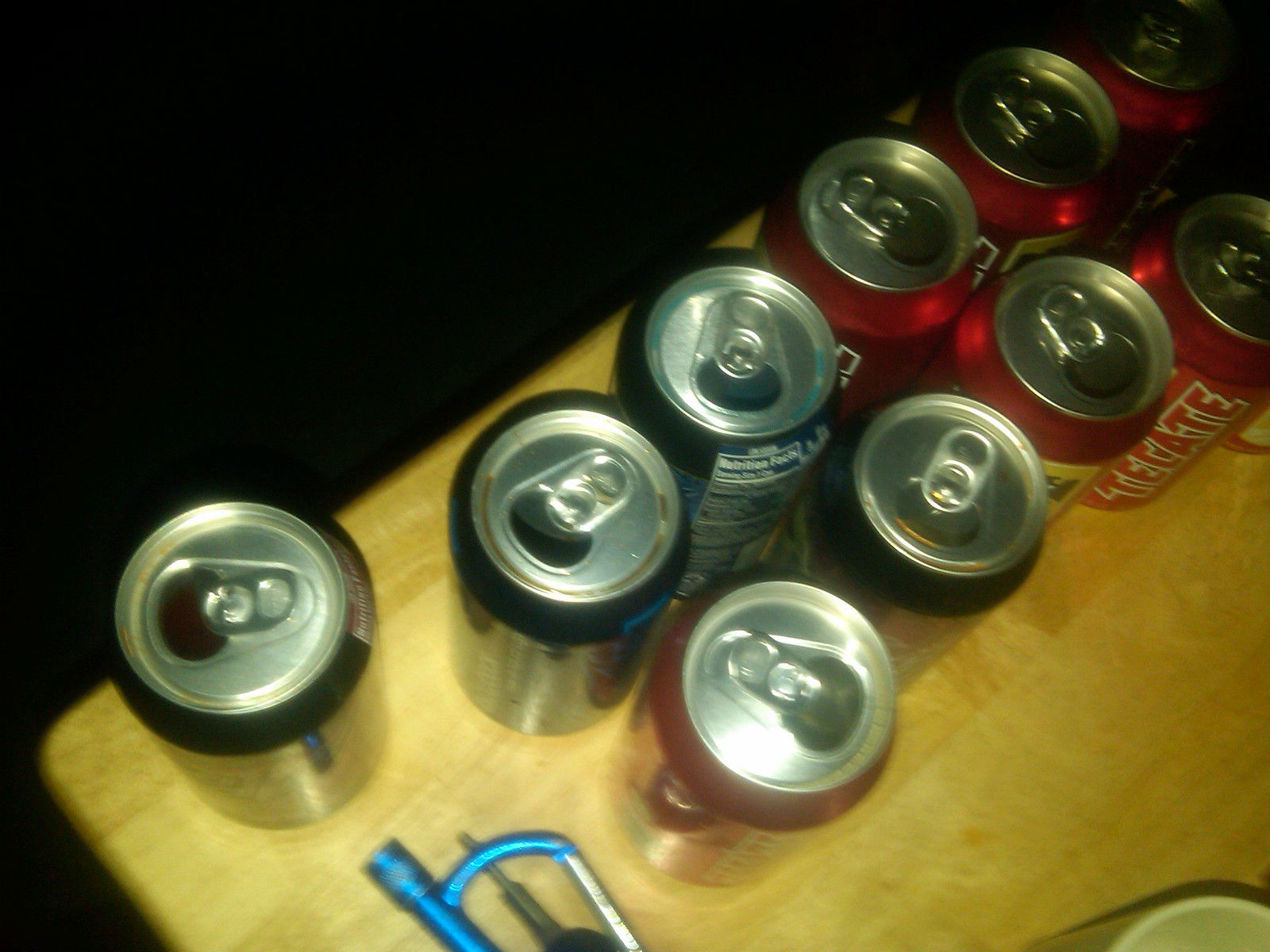This overhead image captures a brown wooden table scattered with a mix of beer cans, predominantly empty and opened. In the arrangement, there are four dark blue cans, which are indiscernible in their specific branding, and six red cans bearing the label "Tecate," a popular beer brand. The placement begins at the left corner with three dark blue cans; the first stands slightly apart from the next two. Adjacent to these are three Tecate cans that extend towards the upper right corner. Below these, another row starts with a Tecate can, followed by a small gap, then one dark blue can, and concludes with two more Tecate cans. An additional Tecate can's triangular section is visible on the far edge. Positioned near the first Tecate can in the second row is a blue carabiner keychain with a single key attached. Additionally, in the bottom right-hand corner lies a segment of a white coffee mug. The composition is well-lit, emphasizing the distinct colors and arrangements of the cans, keys, and cup.